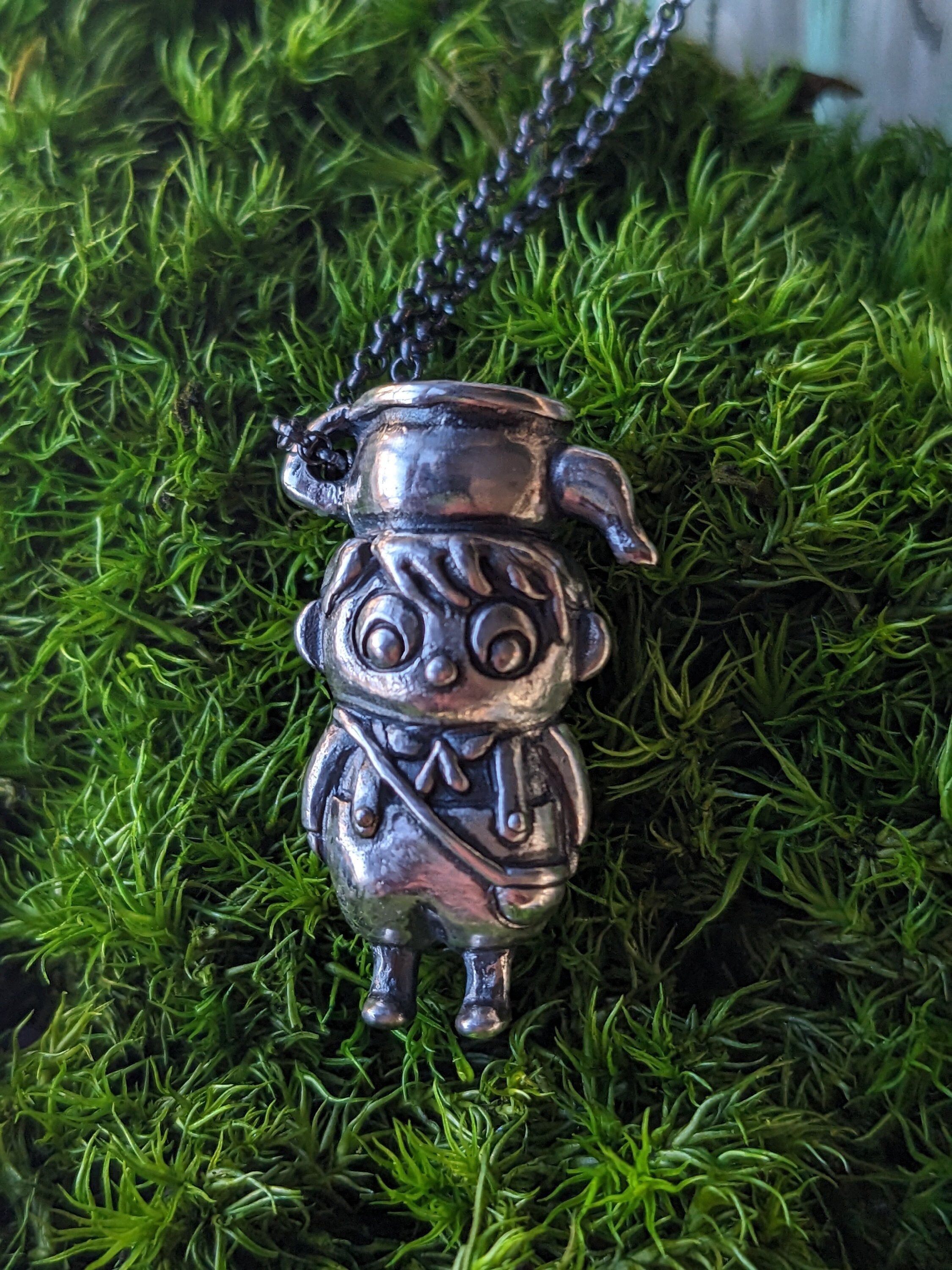This image features an intricately designed metal knick-knack resembling a whimsical little boy. The figure is adorned with a pot or kettle atop its head, characterized by its rosy silver hue. The boy sports endearing features such as large, round eyes and a small, button-like nose. Draped across his chest and shoulder is a miniature purse, while his attire includes suspenders and pants. The knick-knack is positioned on a lush, green grassy base, adding a contrasting natural element to the metallic figure. Additionally, a chain extends from the top of the boy's head, securely attached to the figurine, possibly intended for hanging or display purposes.